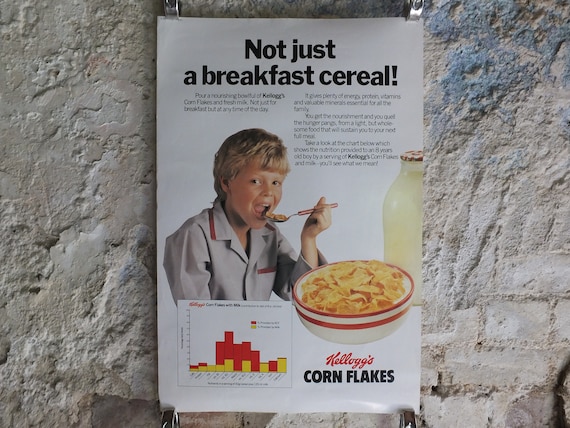This image captures a poster advertisement for Kellogg's Corn Flakes, affixed to a cream-colored, rough-textured wall with metal clips on each corner. The top of the white rectangular poster features the bold black text, "Not Just a Breakfast Cereal," followed by smaller text explaining the nutritional benefits of Corn Flakes with milk, emphasizing its energy, protein, vitamins, and minerals. Below this text, there is an image of a blonde-haired boy eating cereal with a spoon, beside a cream-colored bowl with a red rim filled with Corn Flakes, and a bottle of milk. The lower left side of the poster displays a chart with vertical lines in red and yellow, showing the nutritional content for an eight-year-old boy from a serving of Corn Flakes and milk. The bottom right of the poster prominently features the red Kellogg's Corn Flakes logo.